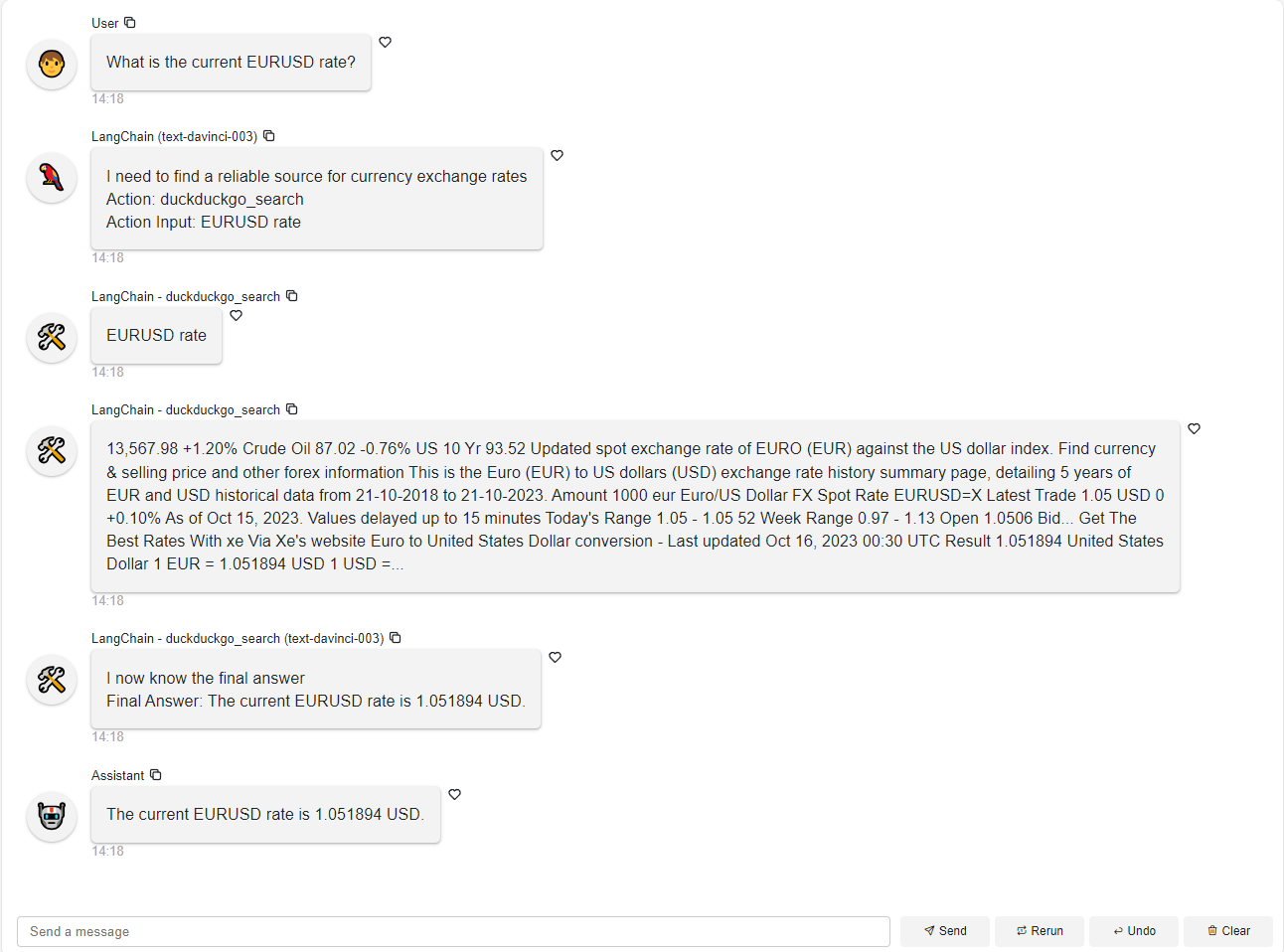A webpage is displayed, resembling an old-school chat room from the early 2000s to early 2010s. The interface features several users posting comments, each with unique, retro, video game-style avatars.

1. **User 1:** An avatar depicting a standard male figure states, "What is the current year USD rate?" Below this message, the number "418" is displayed.
   
2. **User 2:** Represented by a red parrot icon, goes by the username "LangChain (DaVinci003)." The text box reads, "I need to find a reliable source for currency exchange rates." Below this, it indicates an action: "Action: DuckDuckGo_search." The input field shows "EURUSD rate for 18" grayed out.

3. **User 3:** Featuring a wrench and hammer crossed, the username is "LangChain_DuckDuckGo_search" with the text "EURUSD rate" in all uppercase. 

4. Subsequent messages from "LangChain_DuckDuckGo_search" with the same wrench and hammer icon contain extensive information. 

5. In a following message, the same user concludes with "Final answer. The current EURUSD rate is 1.051894 EURUSD."

6. **Assistant:** A user with a transformer head icon confirms, "The current EURUSD rate is 1.051894 EURUSD." 

The detailed exchange underscores the search for accurate currency exchange rates within a nostalgically designed chat room platform.